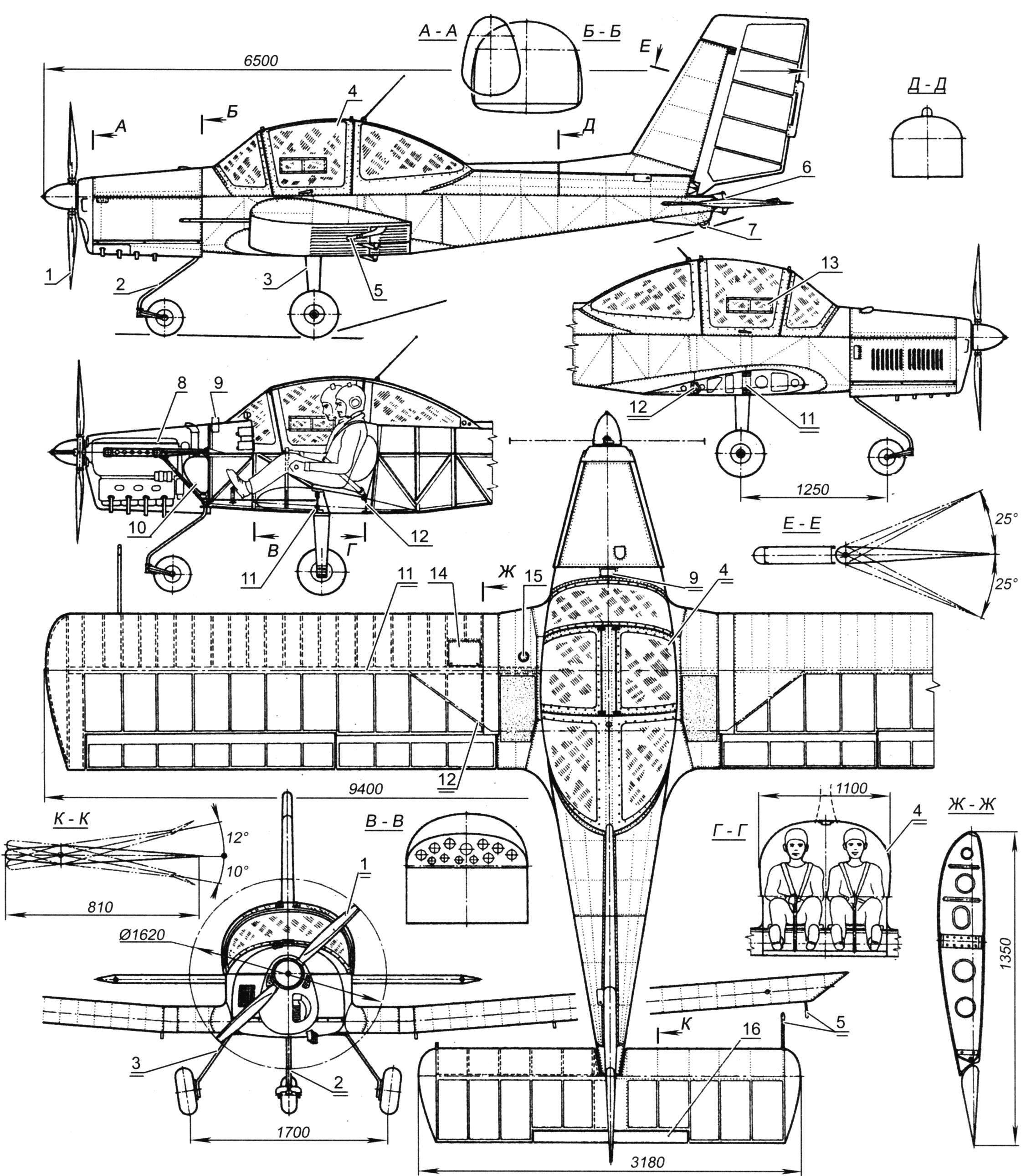The image portrays a detailed engineering schematic of a single-engine aircraft, drawn in black and white with various shades of gray. The diagram includes multiple views and detailed measurements of the airplane. 

At the top is the side profile of the entire aircraft, displaying the propeller at the front and lines indicating its dimensions and shape. Below this side profile is a detailed view of the cockpit, showing two passengers seated near the front. To the right side of the cockpit detail is another side profile focusing on the engine.

Continuing downward, there is a top-down view of the aircraft, highlighting its wingspan and other top features. Below this are the front views: one showing the aircraft’s external front profile and another focused on the front view of the passengers inside the cockpit.

The layout of the illustrations may appear scattered, giving it a blueprint-like appearance devoid of readable text and centered elements, but rich in engineering details and annotations.